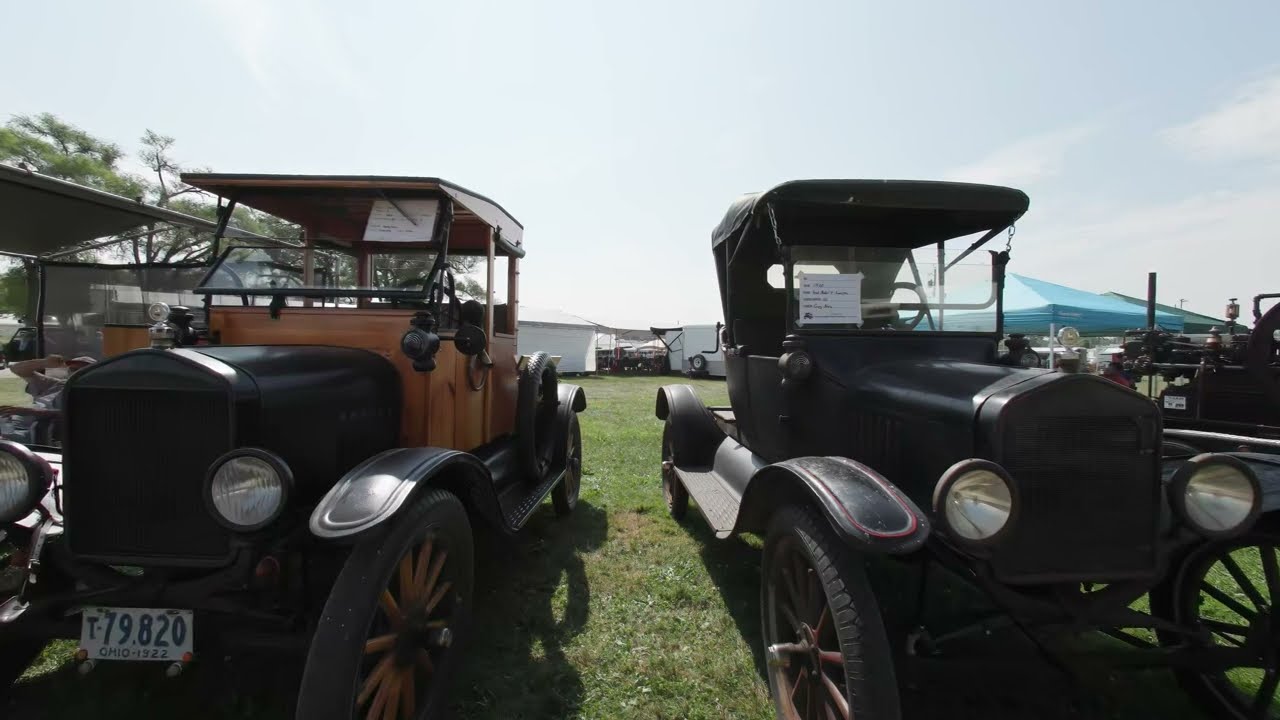This image depicts an antique vintage auto show set outdoors on a grassy surface under a clear, whitish-blue sky. Dominating the center of the scene are two meticulously restored cars from the 1920s, both facing the camera with their grills prominently displayed. The car on the left features a combination of a black front and hood, a striking copper-colored body, spoke wheels, circular headlights, and a distinctive Ohio license plate reading "T79820, 1922." Meanwhile, the car on the right is entirely black, also equipped with spoke wheels and twin round headlights. Surrounding these vintage beauties, the scene extends to reveal additional antique vehicles set among vibrant green trees, a blue tent, and scattered groups of people, reinforcing the lively atmosphere typical of a farm fair or outdoor car exhibition. The detailed setting, coupled with the diverse yet harmonious color palette of light blue, gray, white, black, tan, brown, and green, captures a nostalgic moment on a perfect summer day.